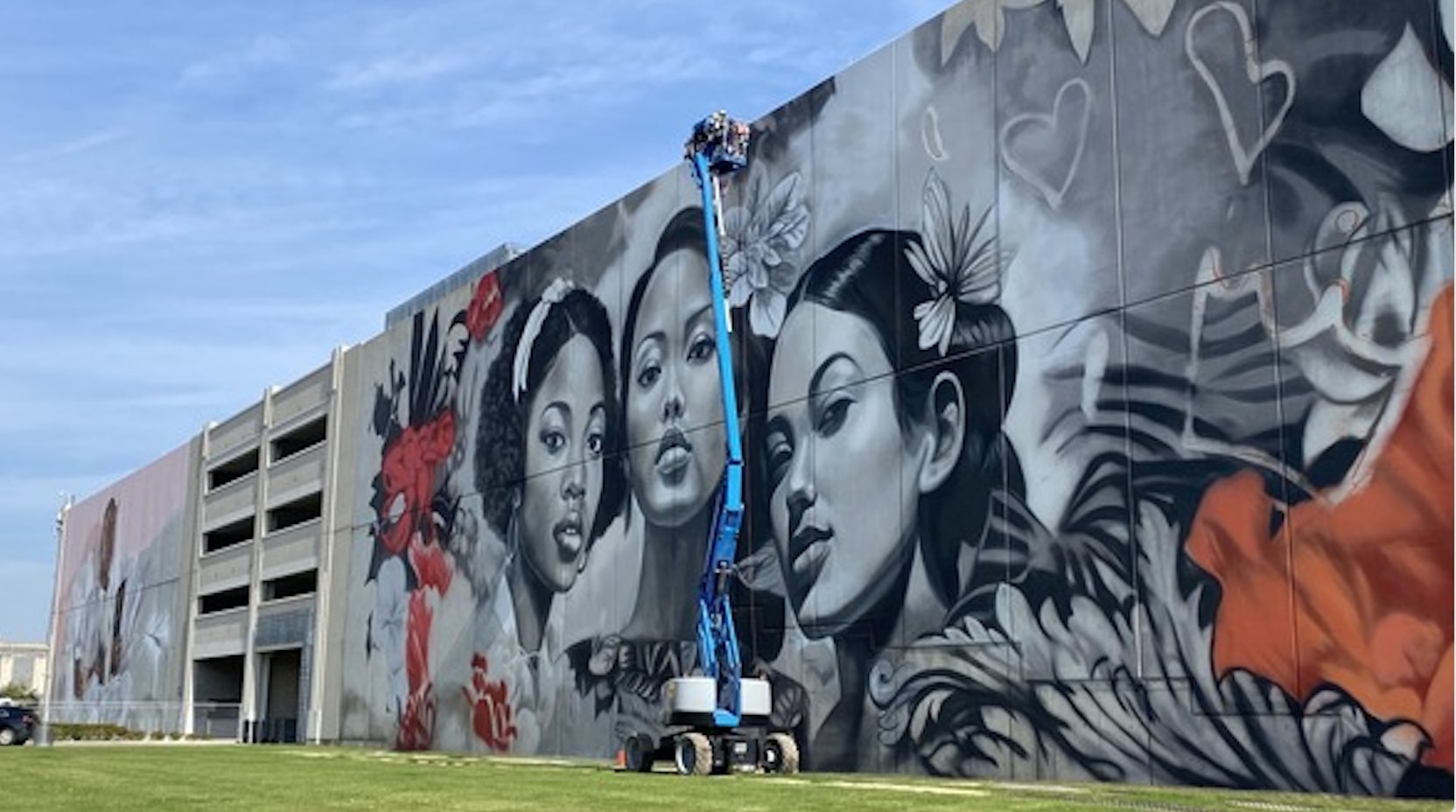The image showcases a stunning, large-scale mural painted on the expansive gray facade of a 5-6 story building, likely a parking structure or warehouse. The mural, which clearly has been officially sanctioned, depicts three strikingly realistic faces of young women from diverse ethnic backgrounds: a Black woman on the left, an Asian woman in the center, and a Latina woman on the right. These faces are intricately detailed in black and white, almost resembling photographs, with vibrant flowers adorning their hair. Surrounding the portraits are abstract elements, including red flowers on the left, heart motifs and leaves on the right, and hints of orange fabric. A freshly mowed grass area lies adjacent to the building, while a blue crane with an artist—indistinguishably male or female—can be seen working on the mural, suggesting it may still be a work in progress. To the left of this primary art, another mural is partially visible. The bright blue sky above completes the scene, emphasizing the mural's grandeur and the vivid colors that contrast with the gray structure.